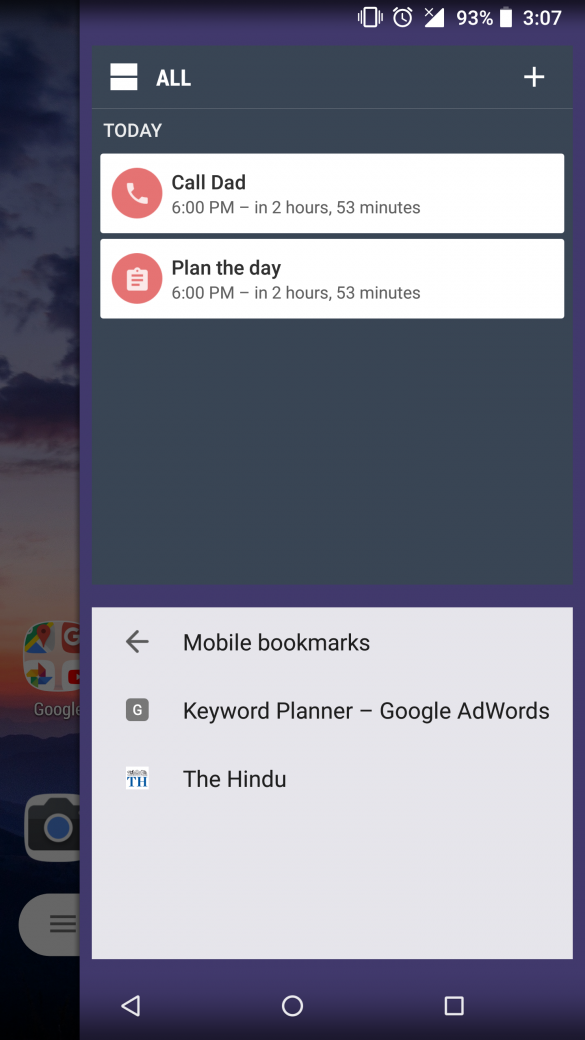The screenshot displays the user interface of a smartphone, predominantly featuring a dark purplish-blue background. At the upper right-hand corner, the time is clearly shown in white text as 3:07, while the battery icon indicates a 93% charge. Additionally, there are icons signifying that the phone is muted and that an alarm is set.

Below this interface on the left side, a headline labelled "All" is visible, followed by the word "Today". Beneath these labels, there are two rectangular cards with slightly off-white backgrounds. 

The top card features a pink phone icon accompanied by the text "Call Dad" in gray font, with a schedule note of "6 PM" and a countdown displaying "In 2 hours 53 minutes".

The second card mirrors this layout but with the text "Plan the day" also scheduled for "6 PM" and the same countdown of "In 2 hours 53 minutes".

At the very bottom of the image, another rectangle with a very light lavender background contains the heading "Mobile bookmarks". Listed below this heading are: "Keyword Planner Google AdWords" and "The Hindu".